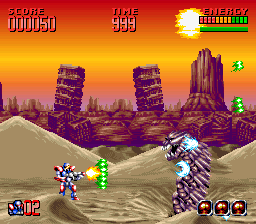In this detailed still from a video game, a vibrant sunset or sunrise casts an orange and pink hue across a desert landscape punctuated by tan sand dunes and brown ruins. Silhouetted against this striking backdrop are leaning buildings on the verge of collapse, adding to the apocalyptic feel. Central to the image is a silver, red, and blue robot-like figure clad in armor. The robot is engaged in a fierce battle, aiming its gun at a monstrous adversary. The gun discharges a vivid blast of orange with hints of green. The menacing monster it targets has a grayish-purple, rock-like body with sharp, white teeth and blue claws resembling crab pincers.

At the top of the image, red font prominently displays a score of "50" and a time of "999." An energy bar beside it features a mix of green, red, and neon green colors. The small details, like the zero-two representation in the corner indicating the robot's attempts or successes, add layers of gameplay depth. This still captures a moment fraught with tension, set against a richly colored sky that transitions from dark orange to twilight hues near the horizon, emphasizing the dramatic and immersive environment.